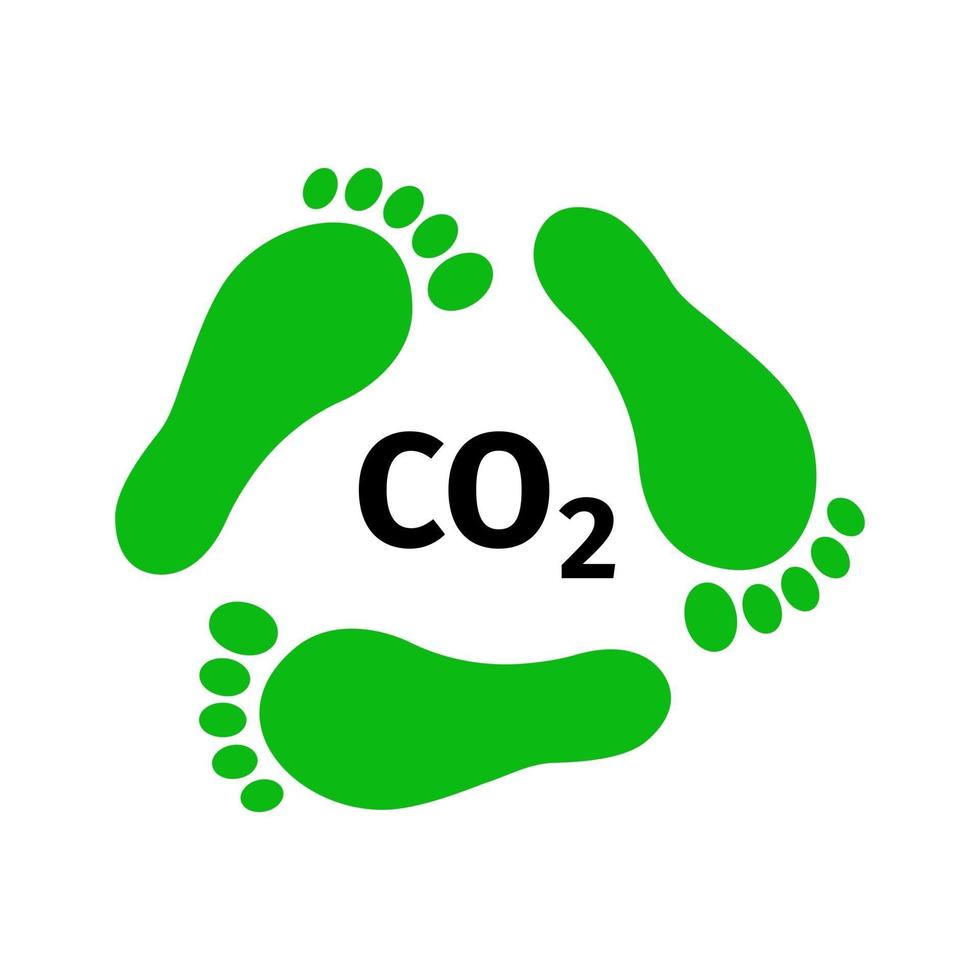The image features a minimalistic design, resembling a branding logo that prominently displays a central text "CO2" in clear and easy-to-read letters, indicative of carbon dioxide. Surrounding the central text are three cartoonish green feet, each with a detailed depiction of the sole and five toes, arranged symmetrically in a triangle shape. The feet, equal in shape and size, appear to be stepping in a clockwise circular pattern. The overall design is reminiscent of environmental symbols, with the green color and the triangle arrangement drawing parallels to the recycling logo, likely implying a message about reducing our carbon footprint to combat global warming.